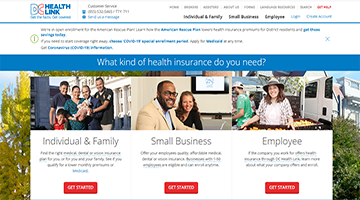Screenshot of the DC Health Link website, prominently displaying options for health insurance categories. The website's name, "DC Health Link," is visible in the upper corner, though a specific web address is missing. The main navigation includes sections tailored to different users: "Individuals and Families," "Small Businesses," and "Employees." Each category features a representative image:

1. **Individuals and Families:** This section displays a family portrait, featuring what appears to be an Asian or Hispanic family with parents and children, including an infant. There's a red "Get Started" button below the image.

2. **Small Businesses:** The middle section shows an African American man with glasses standing beside a white woman with brown hair, both in an office setting. Below the image is another "Get Started" button.

3. **Employees:** The final section captures a white woman with brown hair wearing a hat, set in an outdoor environment that resembles a fair or food truck event. A man in a green shirt and white cap is also partially visible. Like the other sections, it has a "Get Started" button.

An exclamation mark and some text are present but difficult to discern. The overall color scheme features blue prominently, particularly for highlighted text such as "What kind of health insurance do you need?" The image layout is clean and user-friendly, emphasizing a straightforward call to action through the red "Get Started" buttons for each category.